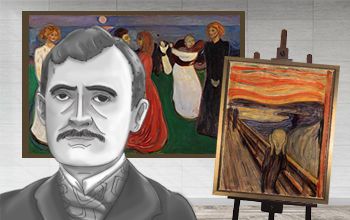The image displays a curated collection of Edvard Munch’s artwork against a light white, wood-paneled backdrop. Dominating the scene is a large painting mounted on the wall, depicting five women in flowing gowns—black, white, red, and white again—dancing on lush green grass with an ocean and a setting sun as their picturesque background. In the foreground, an easel prominently holds a reproduction of "The Scream," showcasing the iconic figure with hands to face, standing on a bridge against a tumultuous sky. Positioned to the left is a detailed black-and-white self-portrait sketch of Munch himself, portrayed in a somber expression, wearing a coat with a distinctive collar and a possible ascot. His mustached visage, with hair styled in a flat wave, gazes thoughtfully out of the image. The floors beneath these art pieces are a variegated gray, adding a neutral contrast to the vivid visual tapestries above.